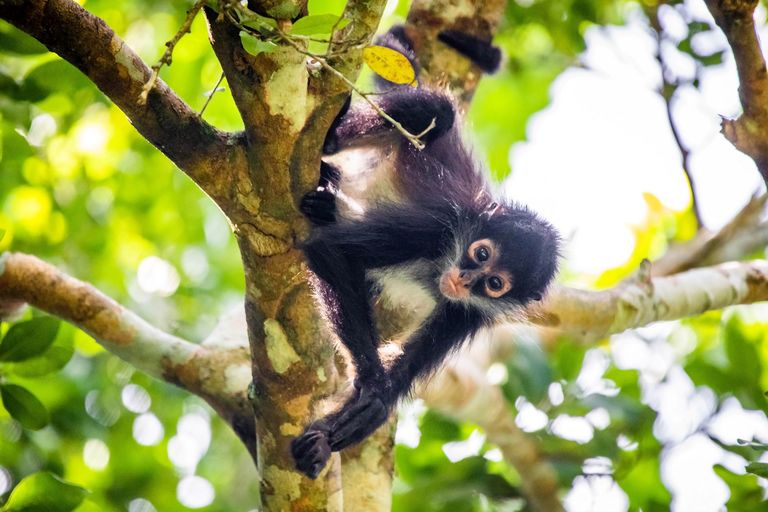In this photograph, we see a small black monkey with a white chest and white facial features, nestled in a tree that suggests a jungle or rainforest setting. The monkey, which appears to be a baby, is hanging partly upside down on a sturdy branch. Its prehensile tail is wrapped around a branch for support, while its long, lanky arms and legs brace it against the tree. The tree, situated on the left-hand side of the frame, has a solid trunk with several horizontally extending branches adorned with green and yellow leaves. Bright sunlight filters through the foliage, creating a vibrant, well-lit backdrop. The monkey has pink skin around its eyes and mouth, and is gazing slightly to the left with no distinct expression on its face. There are no other animals or distracting elements in the image, allowing the viewer to focus on the intricate details of the monkey and its natural environment.